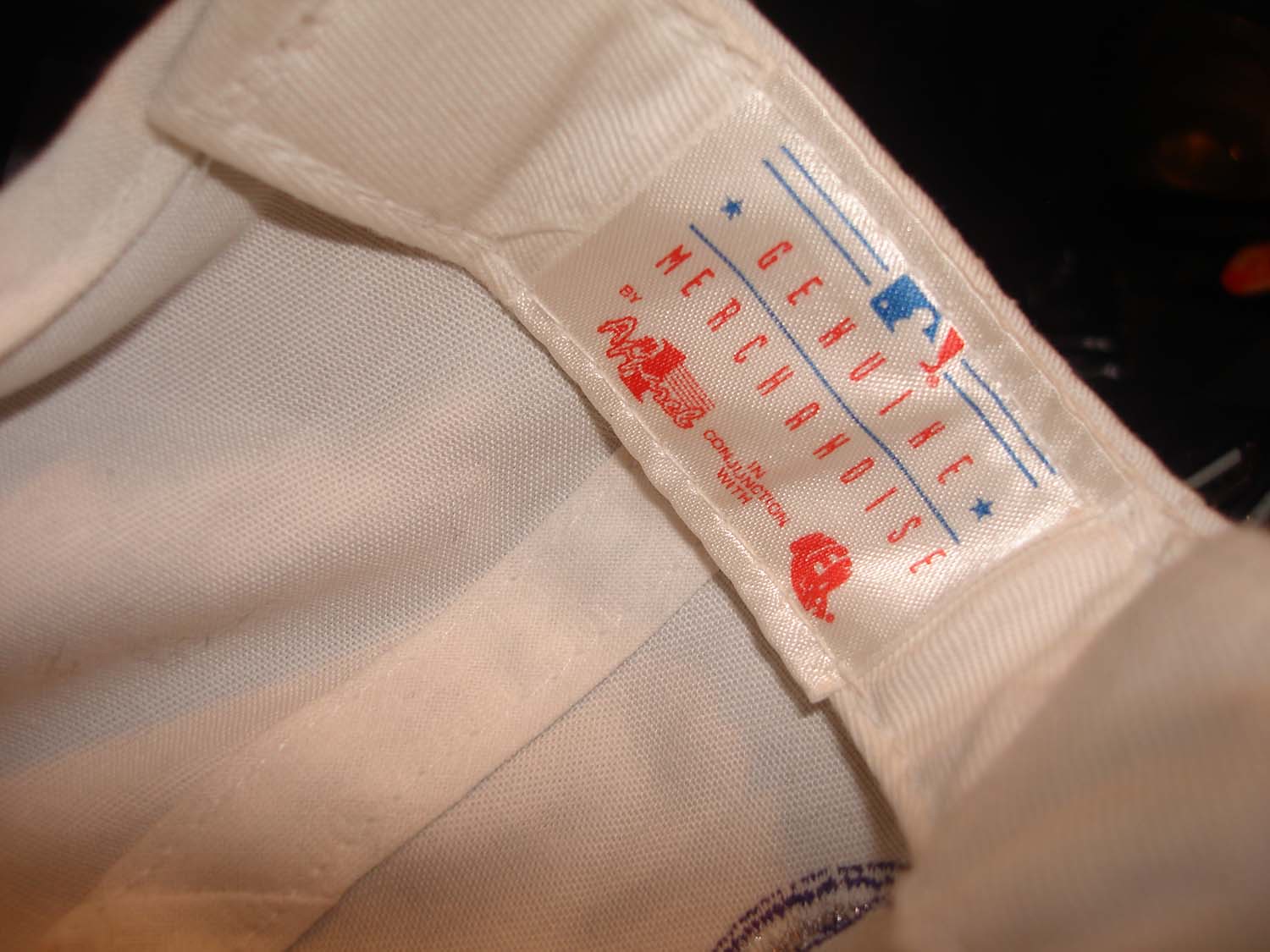This image showcases a piece of clothing, specifically an athletic garment, which appears to be made from exercise-friendly material. The garment is primarily white, with a small black mark located at the bottom middle right-hand side. The focus of the image is on the inner label of the garment. The top of the label prominently features the Major League Baseball (MLB) logo. Beneath the logo, two words are displayed, one directly above the other: "Genuine Merchandise".